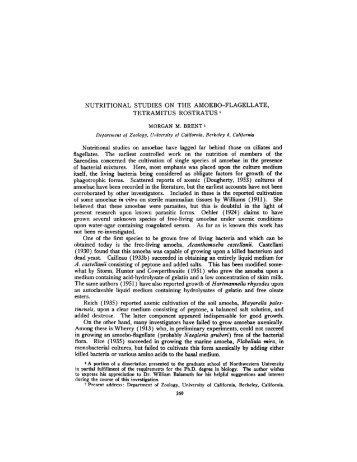The image depicts a very low-quality, blurry, and shadowed scan of a document, making it difficult to read. The document appears to be a small rectangular excerpt, likely from a book page, about one and a half to two inches tall and about an inch to an inch and a half wide. The header, written in large bold print, is clearer and readable, stating "Nutritional Studies on the Amoebo-Flagellate Tetramitus Rostratum." Below this header, the document lists "Morgan M. Brent, Department of Zoology, University of California, Berkeley, California." The main body consists of a lengthy, illegible paragraph in a very small font, possibly including 4 to 6 different types, indicating the complexity of the document. The writing in the paragraph is extremely difficult to decipher, tangibly stating something about nutritional studies lagging behind something else and controlled works in the context of unspecified numbers. There is also a barely discernible page number at the bottom center of the document.